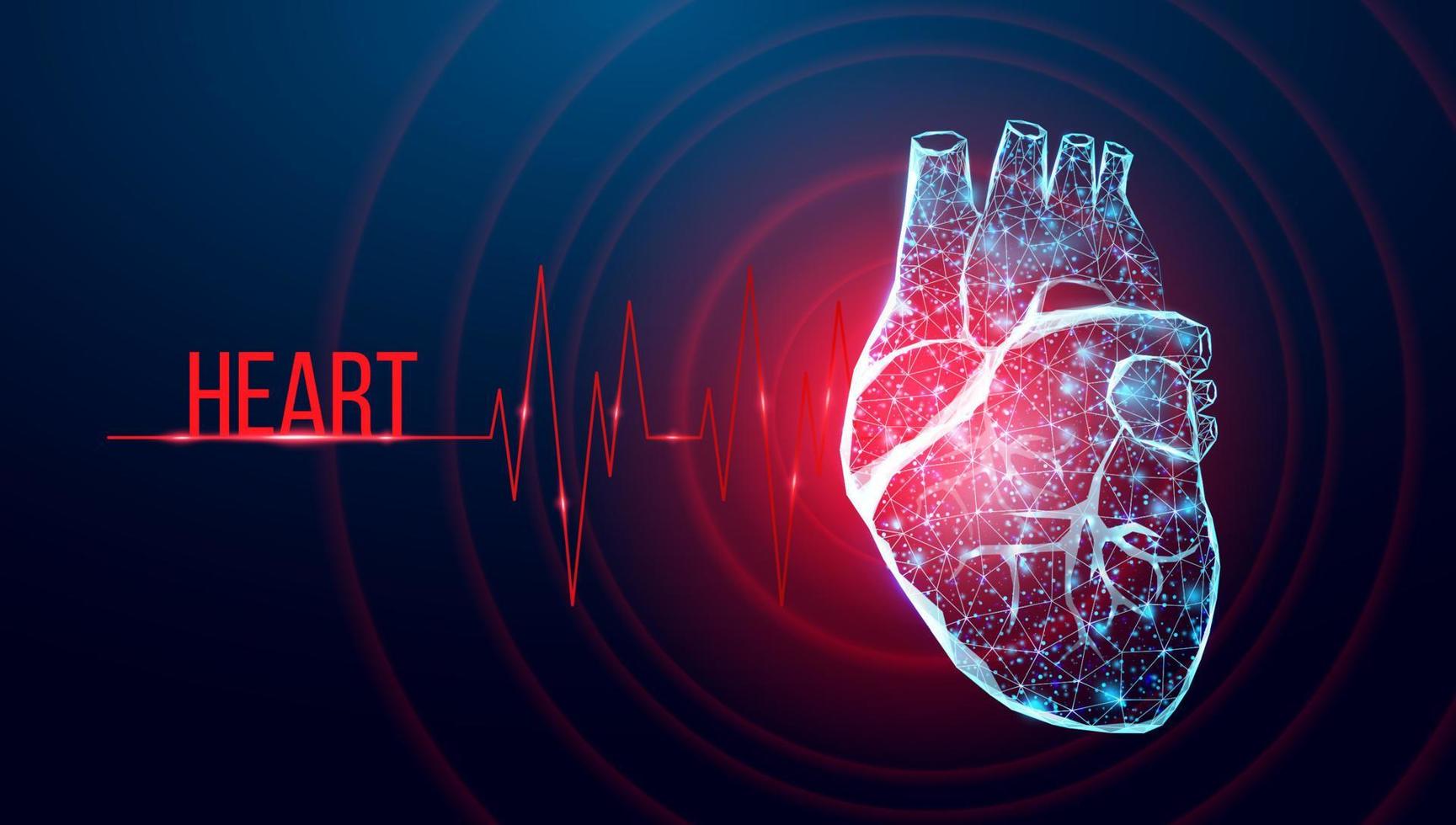This image is a detailed and futuristic illustration of the anatomical human heart. The heart is depicted in a white, translucent style with a cubism-inspired triangular grid overlay. Through its semi-transparent design, some of the internal vessels are visible, adding depth and anatomical accuracy. Surrounding the heart are concentric red circles, emitting from it like sound waves. To the left side of the heart, the word "HEART" is displayed in bold red text above a line that starts straight and then transitions into peaks and valleys, reminiscent of a heartbeat monitor reading. This entire scene is set against a dark, almost black background, giving the image a modern, almost digital feel.